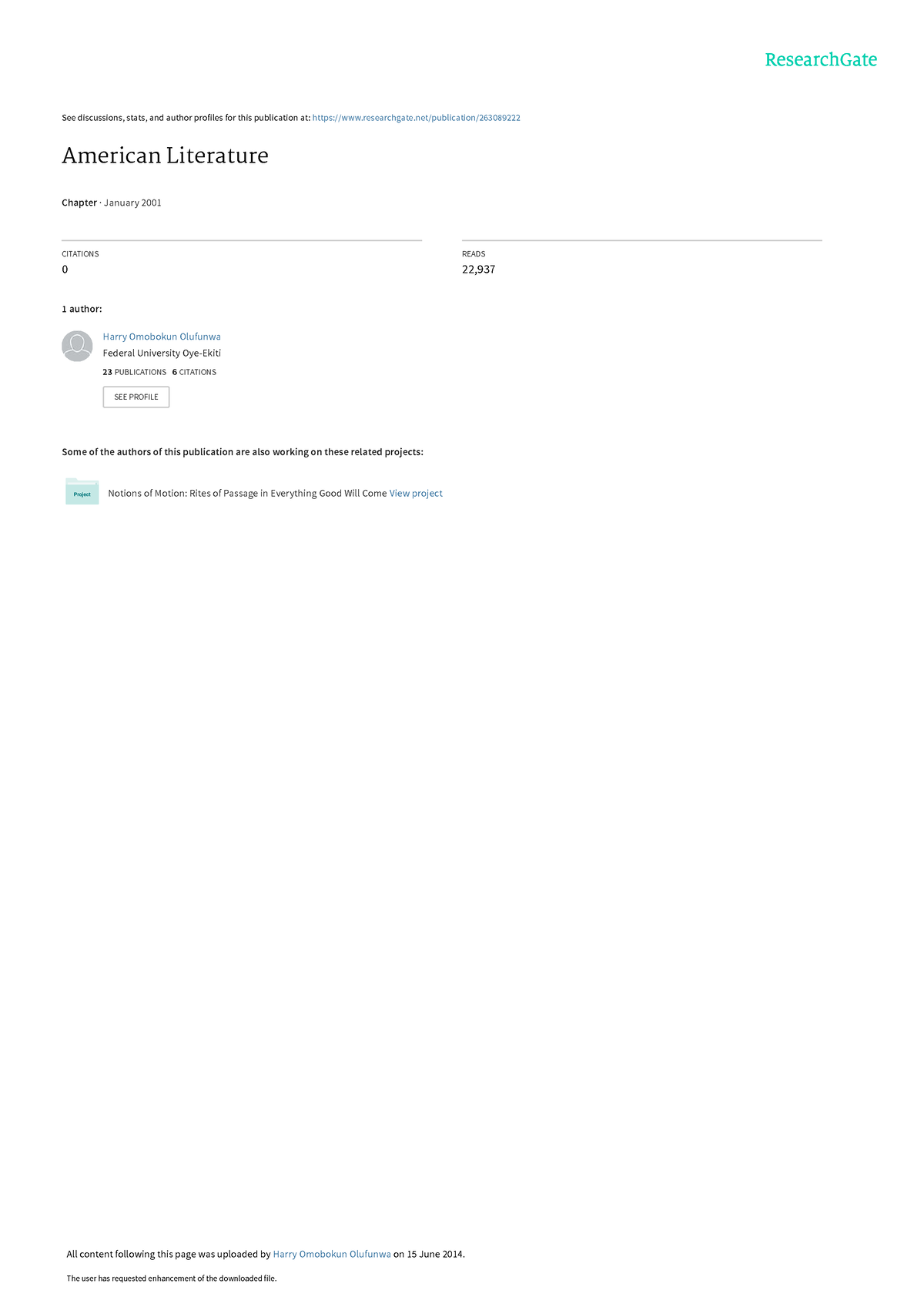The image appears to be a screenshot from the ResearchGate website. In the top right corner, "ResearchGate" is displayed in aqua font. Below this, text in black reads, "See discussions, stats, and author profiles for this publication at," followed by a blue hyperlink that includes "researchgate.net/publication/" and a sequence of numbers which are not fully clear.

Prominently featured in large black medieval-style font is the title "American Literature." Beneath this, in smaller bold black font, it says "Chapter," followed by "January 2001" in a lighter gray font. A faint gray horizontal line acts as a divider below this text.

Next, the word "CREATIONS" is written in all capital letters. Directly underneath, the number "0" is shown in bold. The phrase "1 author:" follows in bold black font, accompanied by a user icon resembling those used on Amazon for users without a profile picture. This icon features a gray background with the white silhouette of a person.

To the right of the icon, the author’s name, "Harry G. Mobokun O. I. Ufunwa," is displayed in blue text. Another faint gray horizontal line separates this section from the following text.

Beneath the second divider, "READS" is written in capital letters, followed by the number "22,937." In the bottom left corner, there is a pale aqua rectangular icon with deep teal writing next to it that reads, "Notions of Motion, Rights of Passage in Everything Good Will Come." Next to this, a blue link text says, "View Project."